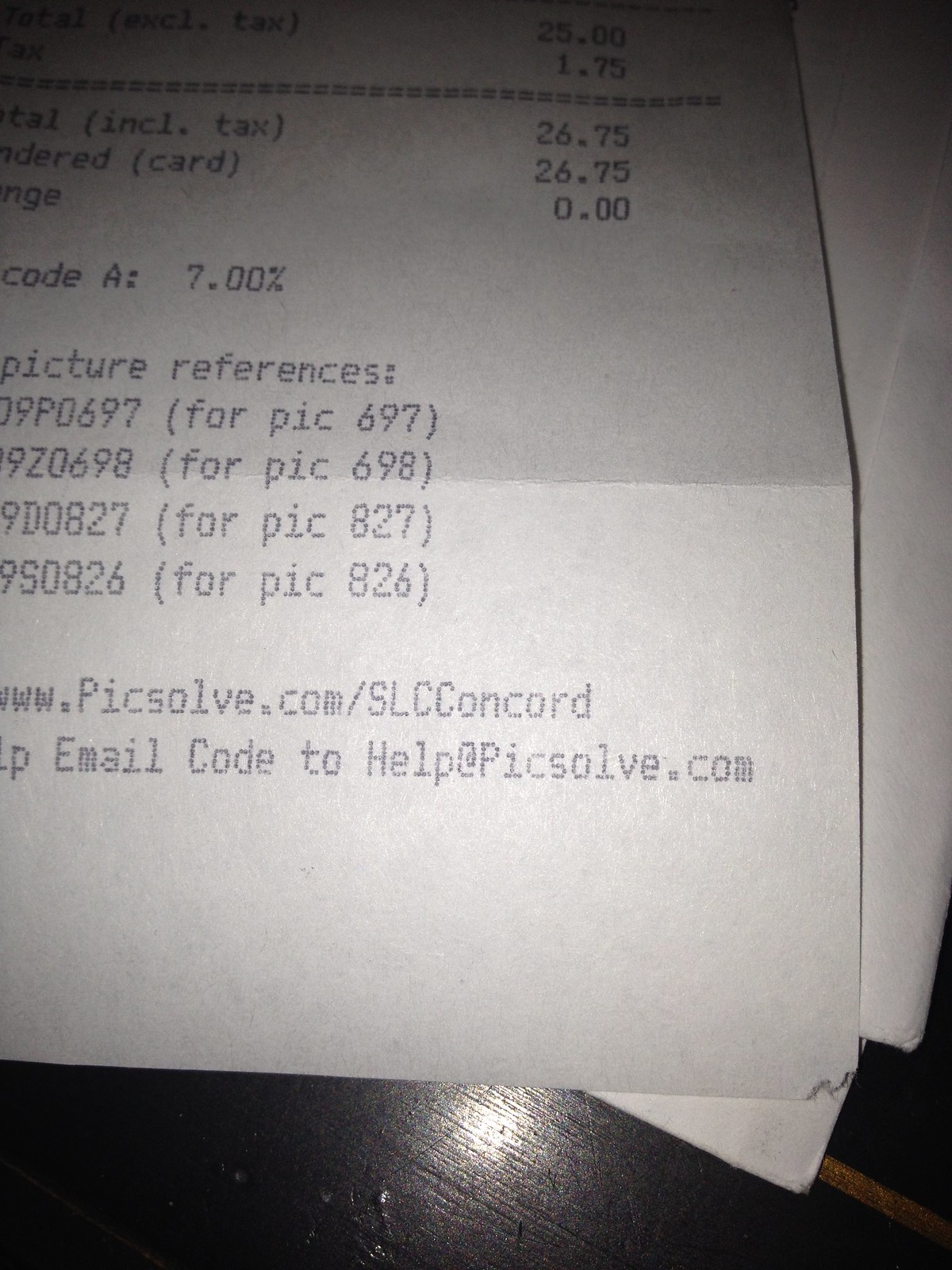Close-up image of the bottom right corner of a receipt from Pixel.com/SLC Concord. The receipt indicates that the customer spent a total of $26.75, likely for a number of photographs. The email address for customer support is provided as help@pixel.com. The receipt is placed among other paperwork and appears to be lined with a shiny black tape, giving the scene a cluttered yet organized look.